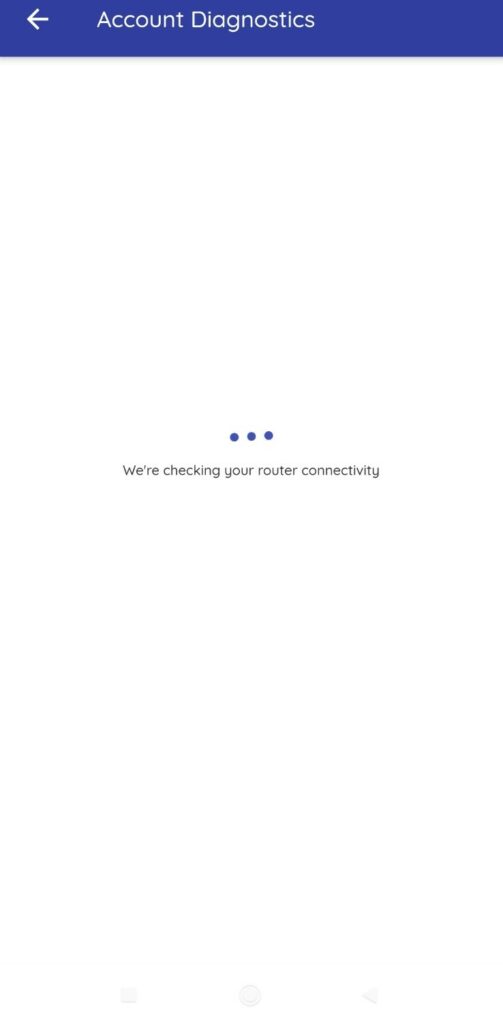This is a screenshot from a mobile device, featuring a predominantly white background. At the very top of the screenshot, there's a bluish-purple bar with the text "Account Diagnostics" centered in white. To the left of this text, there's a white arrow pointing left, indicating a navigation option to go back to a previous page. Below this bar, the screen is largely empty and white, except for a set of three small, purplish-bluish dots arranged horizontally. Beneath these dots is a small line of black text that reads, "We're checking your router connectivity." The lower portion of the image is also empty, with no additional text or elements present. This interface seems to be part of a diagnostics page, likely used for checking the status of the device's Wi-Fi connectivity to ensure there are no issues.